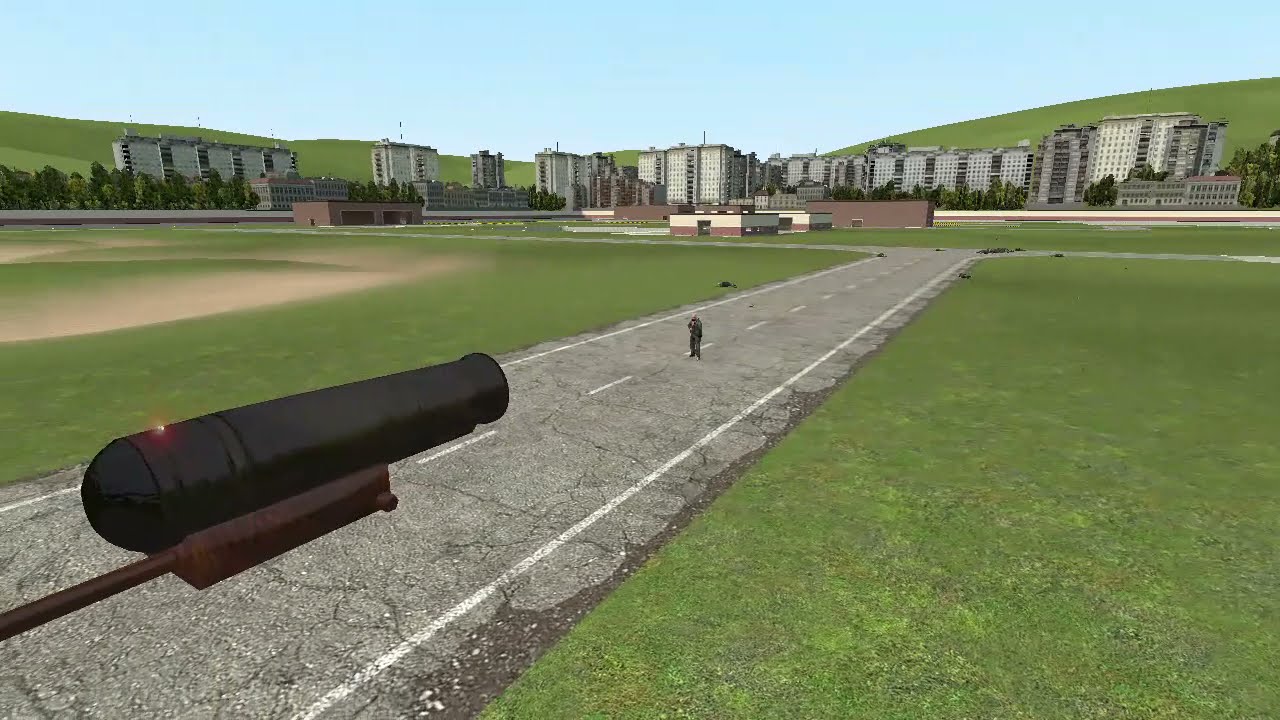The screenshot, taken from a video game, depicts a vast grassy field stretching into the distance. Central to the image is an aged, two-lane pavement road that extends obliquely from the bottom left corner towards the backdrop. This road, reminiscent of an airport runway with a dotted white line down its center, leads towards a cluster of multi-level city buildings nestled before green hills. A lone humanoid character, possibly a soldier, stands approximately 50 to 60 feet away in the middle of the road. Dominating the foreground is a large cannon with a black barrel, mounted on a brown wooden platform, devoid of wheels and supported by a rusty arm, positioned close to the bottom left, pointing towards the character. Despite the seemingly serene landscape, the low-quality graphics and the unusual placement of the cannon and character add a layer of mystery and intrigue to the scene, framed by a clear blue sky overhead.